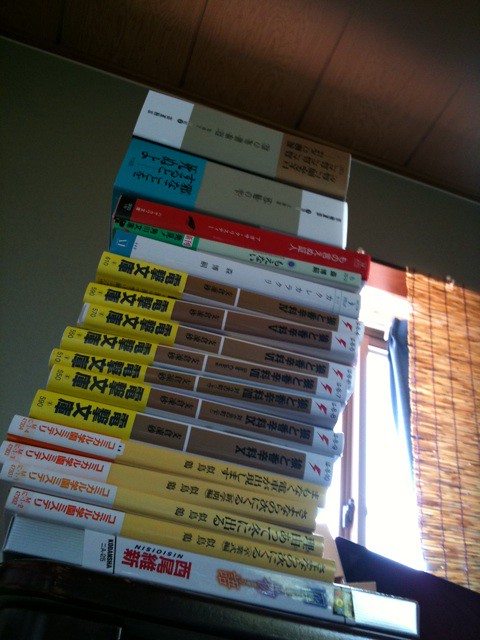The photograph captures a dimly lit interior of a house, focusing on a towering stack of books arranged horizontally on top of each other. The angle of the shot, taken from below, makes the books appear even taller. The right side of the image is brightened by glaring white light streaming through a window, which is covered by a bamboo roll-up shade. The space has a drop ceiling, evident from the visible outlines of ceiling tiles. The stack consists of around 15 books, all in Japanese, ranging in color and format. The base of the stack features a white-spined book, possibly a hardback. Above it, four paperback books have white spines with red and yellow lettering. Following those are seven books from the same series, each with a yellow and brown spine adorned with black text. Additional larger books top off the stack, including one with a tan and green spine, and another with a red spine. The two books at the top appear chunkier, possibly encased in slipcovers commonly used in Japan. The varied colors and styles of the spines, combined with the distinct foreign characters, create a visually intriguing and culturally rich focal point amid the warm, ambient setting of the room.